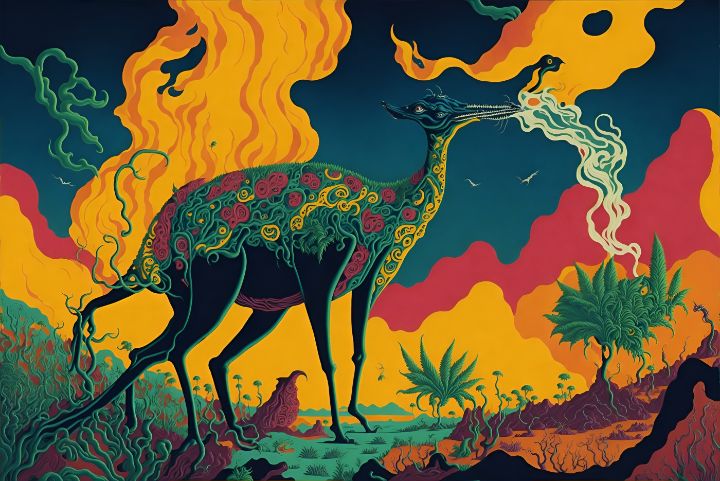This is an artistic, somewhat abstract painting presented in a horizontally aligned rectangular format without a border. Dominating the center of the image is a fantastical creature that combines features of different animals: it has a small head with a narrow, sharp beak resembling a bird or dinosaur, set atop a large, colorful body. The creature's body is a swirling mosaic of green, pink, orange, red, yellow, and black hues with thin, black limbs and a distinctive, slender tail. Emanating from its mouth are flame-like wisps, though unusually colored in white.

The painting’s vivid backdrop suggests an open, expansive landscape, potentially an African safari-like desert rather than a jungle. The background is rich and dynamic, portraying a night sky in dark blue and black tones interspersed with vertical orange curves hinting at flames or sand dunes. Along the bottom are brighter greens symbolizing land, and to the right, a small green bush. The horizon features reddish and yellowish mountain-like shapes, further intensifying the landscape's abstract yet vibrant quality. Scattered gray birds add an element of depth and animation, enhancing the painting's colorful and lively atmosphere.